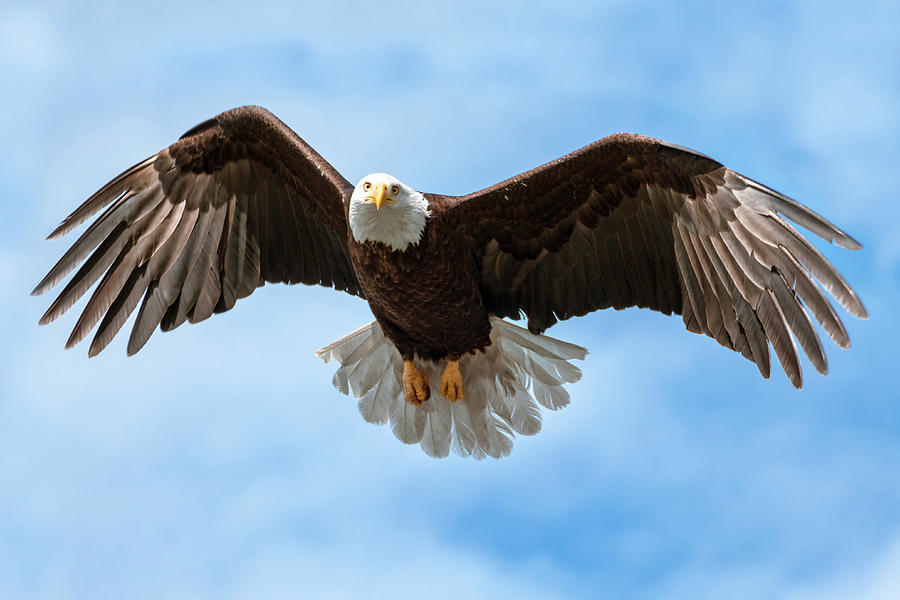The image depicts a majestic bald eagle in mid-flight, its powerful wings, brown with lighter tips, fully outstretched from left to right. The eagle is oriented towards the right of the image, its white-feathered head, sharp yellow beak, and orange talons clearly visible. Its white tail is fanned out, contrasting with its body. The background features a serene blue sky dotted with wispy white clouds, which is blurred to keep the focus entirely on the bird. The composition almost resembles a painting or an AI-generated image due to its striking clarity and aesthetic appeal. The bald eagle's intense gaze is captured as it soars, making it the sole and captivating subject of the photograph.